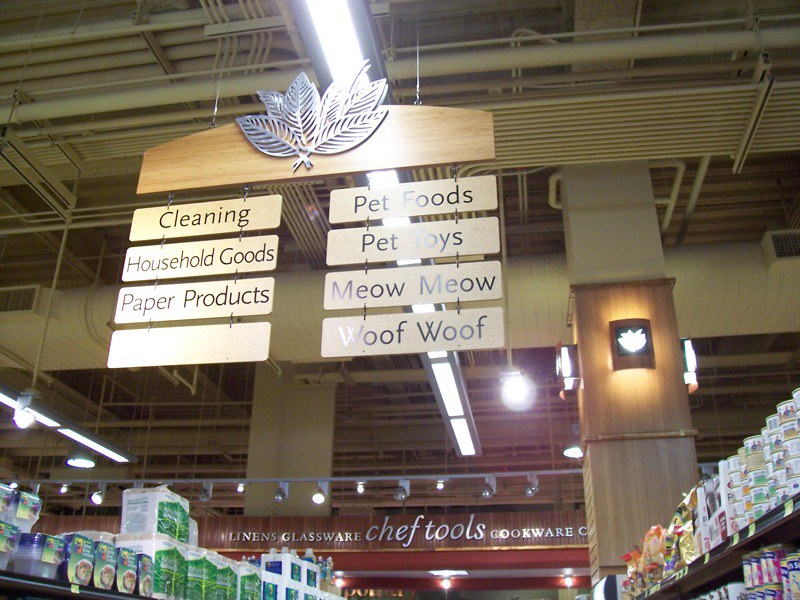The photograph captures a detailed view inside a supermarket aisle, with the camera angled upward to center on a hanging aisle sign. The sign, made of a piece of maple wood adorned with cut-out silver metal leaves, features two columns of placards listing the aisle's contents. In the left column, the placards read "Cleaning," "Household Goods," "Paper Products," with the bottom placard blank. The right column lists "Pet Foods," "Pet Toys," “Meow Meow,” and "Woof Woof." The background reveals the far wall of the supermarket, which has additional signage reading "Linens," "Glassware," "Chef Tools," and "Cookware" in white lettering. The ceiling, visible toward the bottom and top of the image, shows exposed metal rafters, piping, and a row of fluorescent lights. Prominently displayed on the top shelves of the aisle are a variety of products, with canned goods on the right and Tupperware containers and paper towels on the left. The photograph is well-focused, giving a comprehensive view of this section of the store.